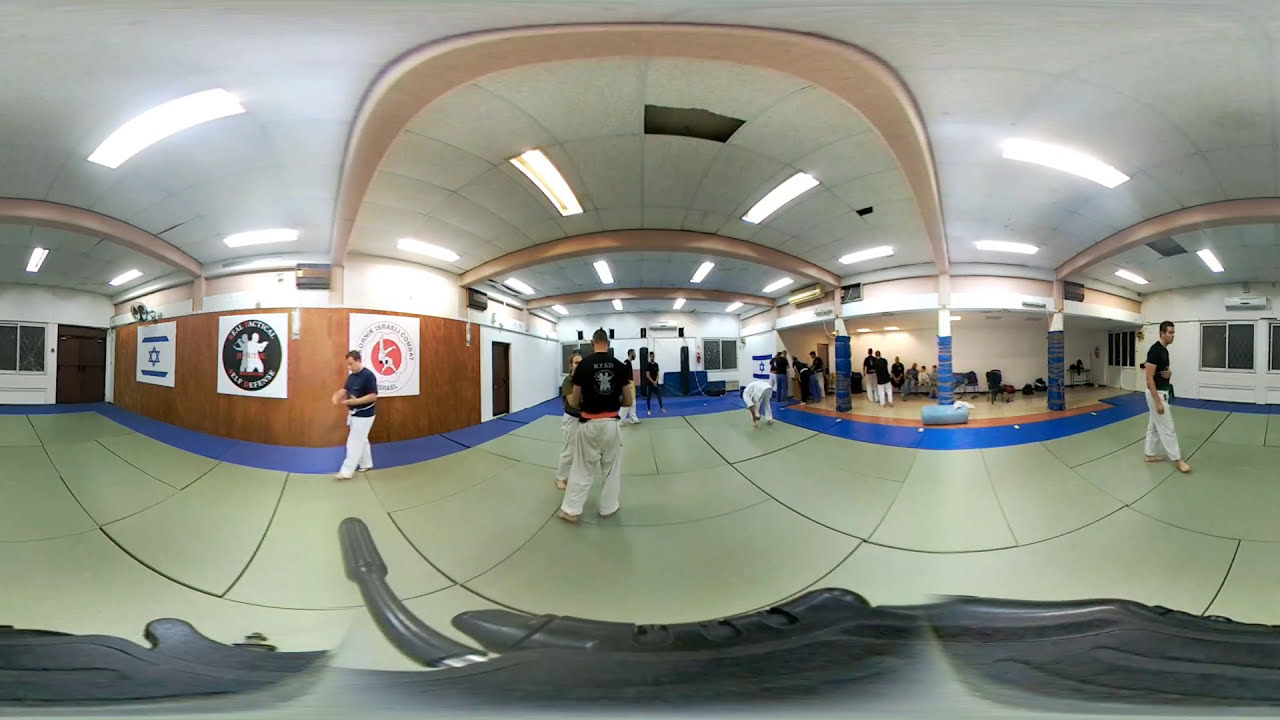The image shows a panoramic view of a karate dojo taken with a fisheye lens, giving it a slightly curved and distorted appearance. At the center stands a man with his back to the camera, dressed in a black t-shirt and loose-fitting white pants, barefoot, with a red belt around his waist. He stands on green padded flooring that curves with the fisheye effect, and in front of him, the floor transitions to blue padding which becomes white at the back of the dojo.

To the left of the central figure, another individual is walking with a black shirt and white pants, head facing down, hands in front. On the far right, a person stands on one foot, with the other foot forward, hands at hips, and black hair. In the background, several other people can be seen, including one in a full white uniform bending over on the blue stripe.

The dojo's interior features a light brown wooden arch on the ceiling, with off-white panels and square cutouts through which a dirty yellowish light filters. The right wall is mostly white with a couple of windows and frames, while the left wall is wooden with banners hanging. These banners have white backgrounds with various symbols: the leftmost has a Star of David, the center one features a black circle depicting people practicing karate, and the rightmost one shows an orange circle with a person performing a karate move.

In the rear, there's a staging area with a wooden floor where people gather to sit or perform additional exercises. Some people are engaged in solo exercises or stretching, wearing either parts of a karate uniform or black shirts and white pants. The overall scene suggests an active martial arts practice session within a well-equipped dojo, possibly in a foreign country as hinted by non-English signs on the walls.